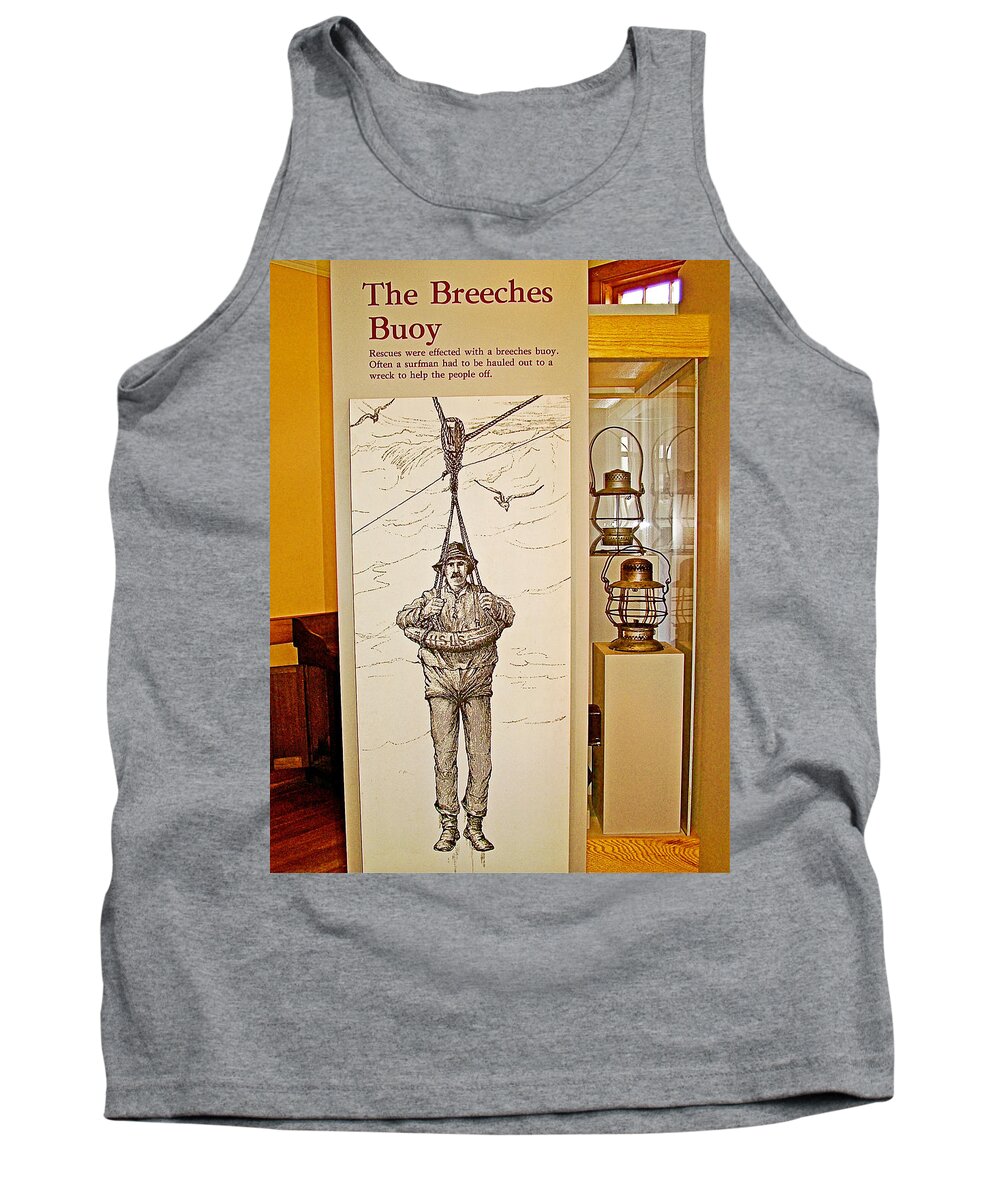The image depicts a simple, light gray tank top with slight wrinkles against a white background. Superimposed onto the tank top is a photorealistic graphic resembling a book cover titled "The Breaches Buoy." Below the title, text explains that rescues were carried out using a breeches buoy, often involving a surfman being hauled out to a wreck to assist stranded individuals. The graphic features a pencil sketch of a man suspended by a rope, wearing a life preserver with attached shorts and full wet weather gear, including a hat. He is depicted dangling with his feet below him. To the right of this sketch, there are two brass lanterns, appearing to be part of a museum exhibit inside a display case. The overall composition blends the simplicity of the tank top with the intricate details of the historic rescue scene and accompanying artifacts.